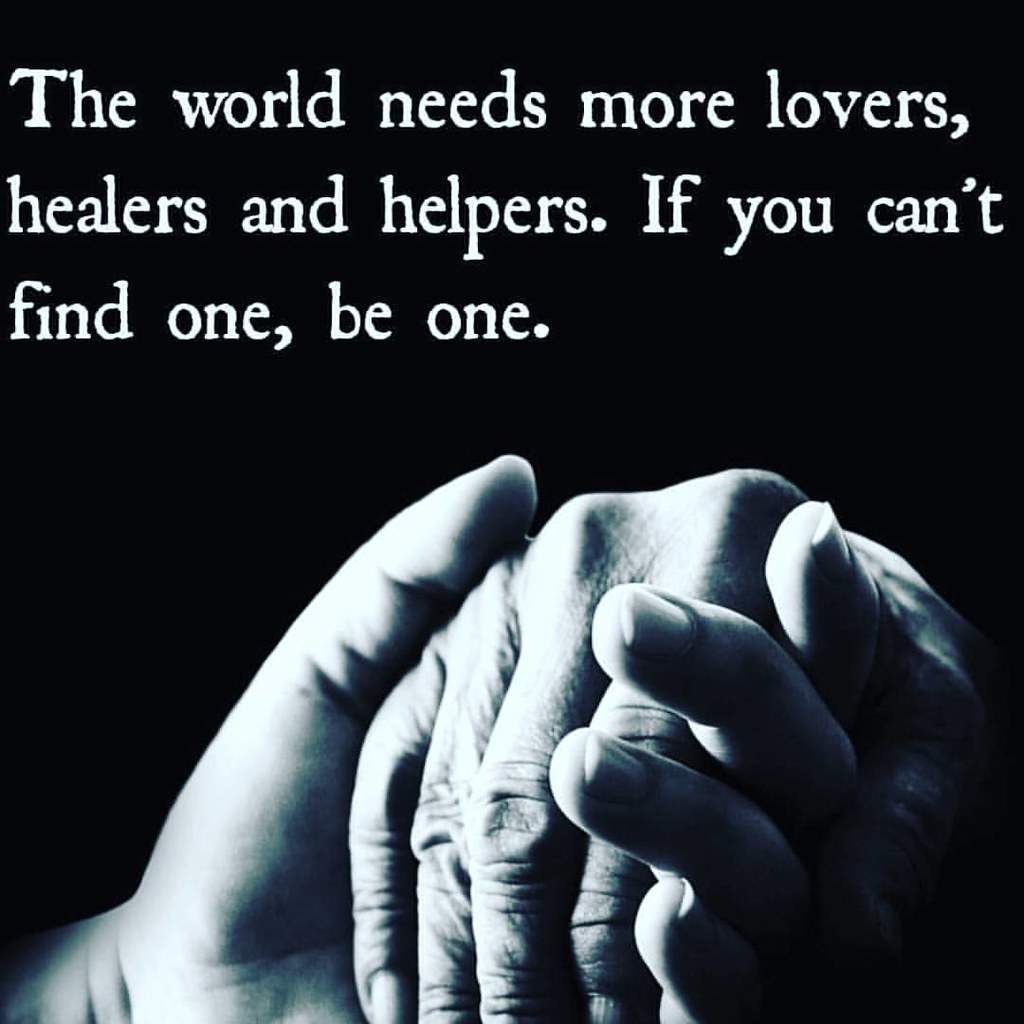The image features an inspirational black and white poster with a completely black background. Dominating the bottom half are two clasped hands—an older, wrinkled right hand gently held from underneath by a smoother, younger left hand. Above this touching scene are three lines of white text in a serif font, reading: "The world needs more lovers, healers and helpers. If you can't find one, be one." The design captures a tender moment of intergenerational connection and emphasizes the importance of compassion and support, with the contrasting textures and ages of the hands highlighting the timeless nature of these values.